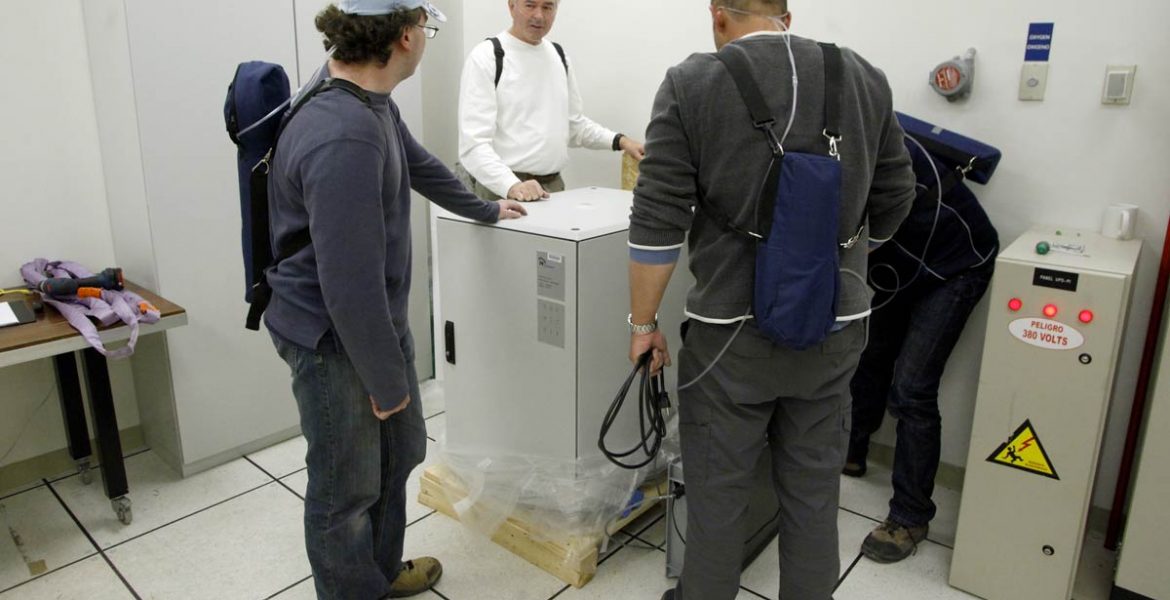The photograph depicts the interior of a brightly lit, white-tiled room, likely in a laboratory or technical setting. Four men are positioned around a metallic, white cuboidal machine that appears to be newly arrived, as it still rests on a wooden pallet wrapped in plastic at the base. The central focus is the machine, which seems related to electrical or medical equipment.

On the far left, a man with curly brown hair, wearing a long-sleeved gray shirt and jeans, is engaging with the machine, his left hand resting on top of it. He sports a backpack with blue straps. Opposite him is another man in a white shirt, his face partially out of the frame, also interacting with the device, with black backpack straps visible over his shoulders. To the right side of the machine stands a man in a rolled-up long-sleeved gray shirt, gray pants, and brown shoes, holding a coiled black cord in one hand. He too wears a blue backpack.

A fourth individual, dressed in black and positioned slightly away against the right wall, is partially visible. The background features additional electrical equipment, including a gray rectangular box with three red lights and a warning label, indicating high voltage, along with a gray cabinet and a small table cluttered with items on the left side of the room.